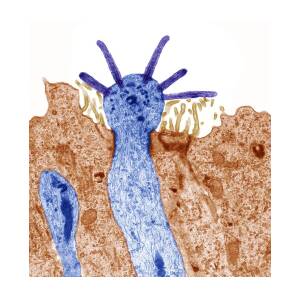The image appears to be a painting, which may either be children's art or possibly a scientific illustration. It is roughly square-shaped, about an inch and a half in both height and width. The background is predominantly white, with the top third of the image left as plain white paper. Below this, there's a peachy-orange or light brown area that resembles uneven dirt or an organic substance with light and dark brown hues. This painting may have been created using crayons or markers, adding to its textured and colorful appearance.

Emerging from the lower part of the painting, predominantly on the left-hand side, there are amoeba-like, single-celled structures. The most striking element is a large blue figure located at the bottom center, extending upwards. It has an elongated, oval body with dark blue detailing on one side and a rounded "head" on top, adorned with five blue or purple hair-like extensions or spikes. This figure is detailed with many dots, where the body is mostly light blue with dark blue accents. To the left of this central structure, there is another smaller blue shape embedded in the background with a similar patterned coloration.

Additionally, surrounding these blue figures, there are several smaller, brown, V-shaped structures. These also have dark brown dots scattered across their light brown bodies. The painting is characterized by its abstract forms and vivid colors, making it a unique and visually engaging piece.